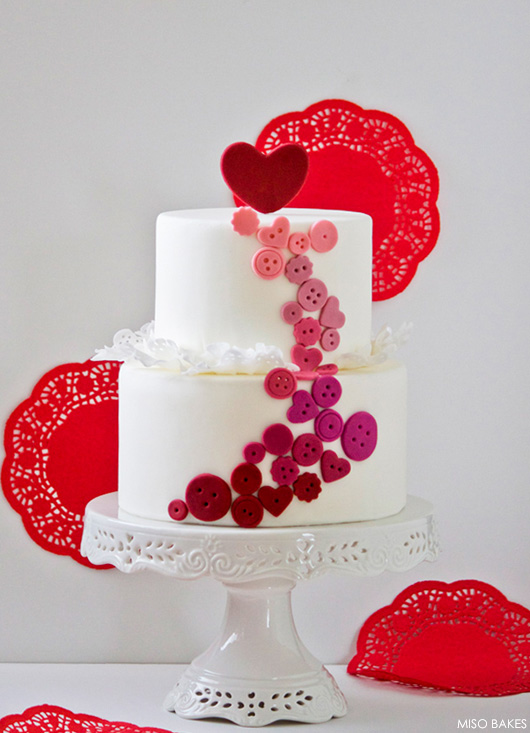This image features a decadent two-layer Valentine's Day cake, prominently displayed on an elegant white porcelain cake stand with intricate holes and swirls at its base. The cake is a pristine white, with the larger bottom layer supporting a smaller top layer, each adorned with a mix of red, pink, and purple fondant hearts extending vertically from the bottom to the top. The topmost highlight is a striking red heart standing upright, adding a festive touch. The cake is placed against a medium gray backdrop, further accented by decorative red circular doilies on the white table and hanging on the wall, enhancing the romantic theme. In the lower right corner of the photo, the words "Miso Bakes" suggest the cake's creator or brand.